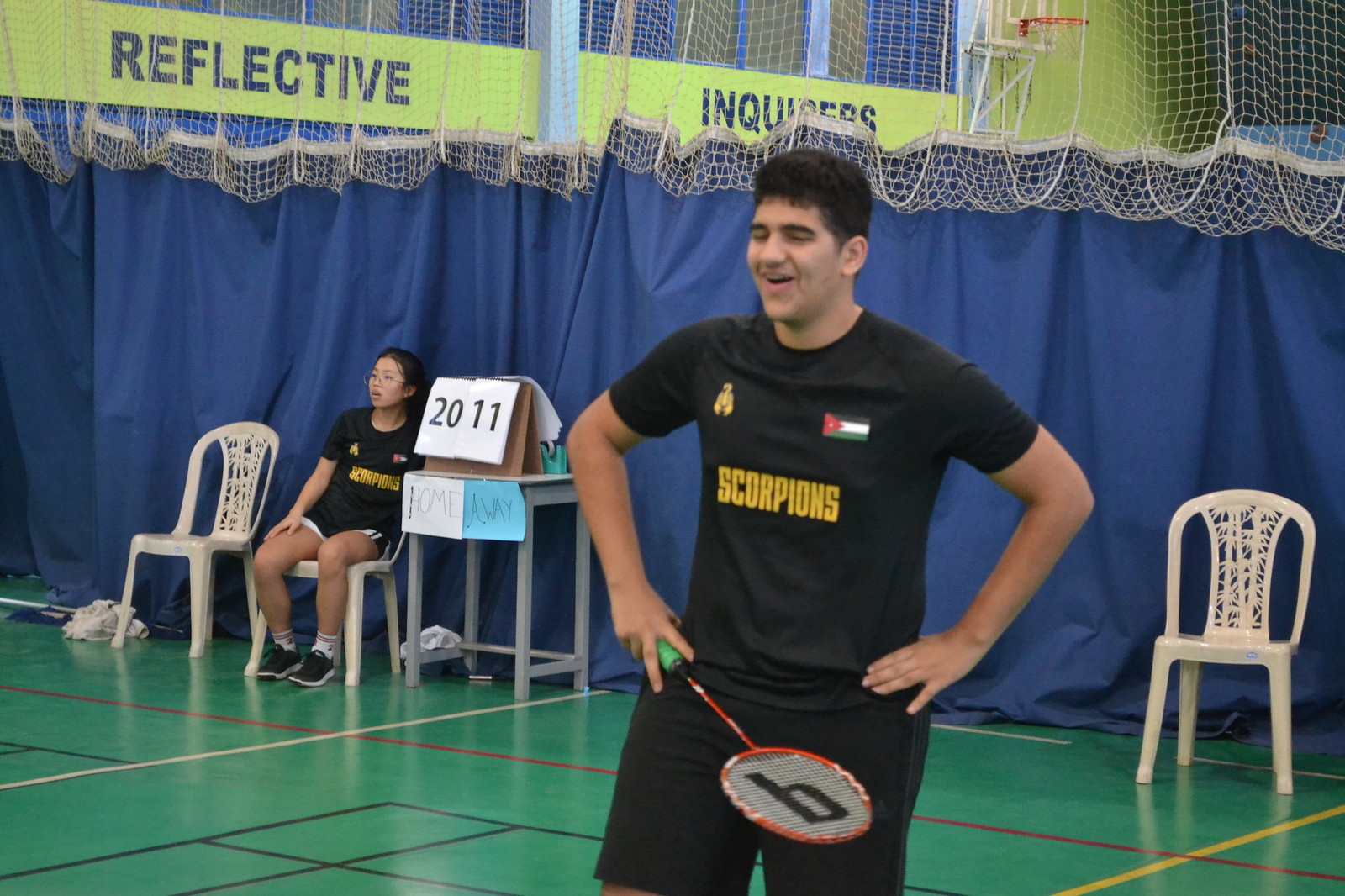A man is photographed at a sporting event, likely a badminton match, as he is holding what seems to be a badminton racket. He is dressed in a black t-shirt and black shorts, with the word "Scorpions" emblazoned in yellow on the shirt. The shirt also features a small flag on the right side of his chest and a yellow emblem on the left. In the background, a woman wearing a similar Scorpions shirt is seated off to the side in an off-white plastic chair beside a table with a sign reading "2011." The setting is indoors, with a shiny green vinyl floor marked with various colored lines outlining the court. A blue curtain, partially see-through due to a mesh net at the top, creates a wall-like appearance, and hints of a basketball court can be seen beyond it. Hanging above, there is a reflective yellow board displaying the word "increase."